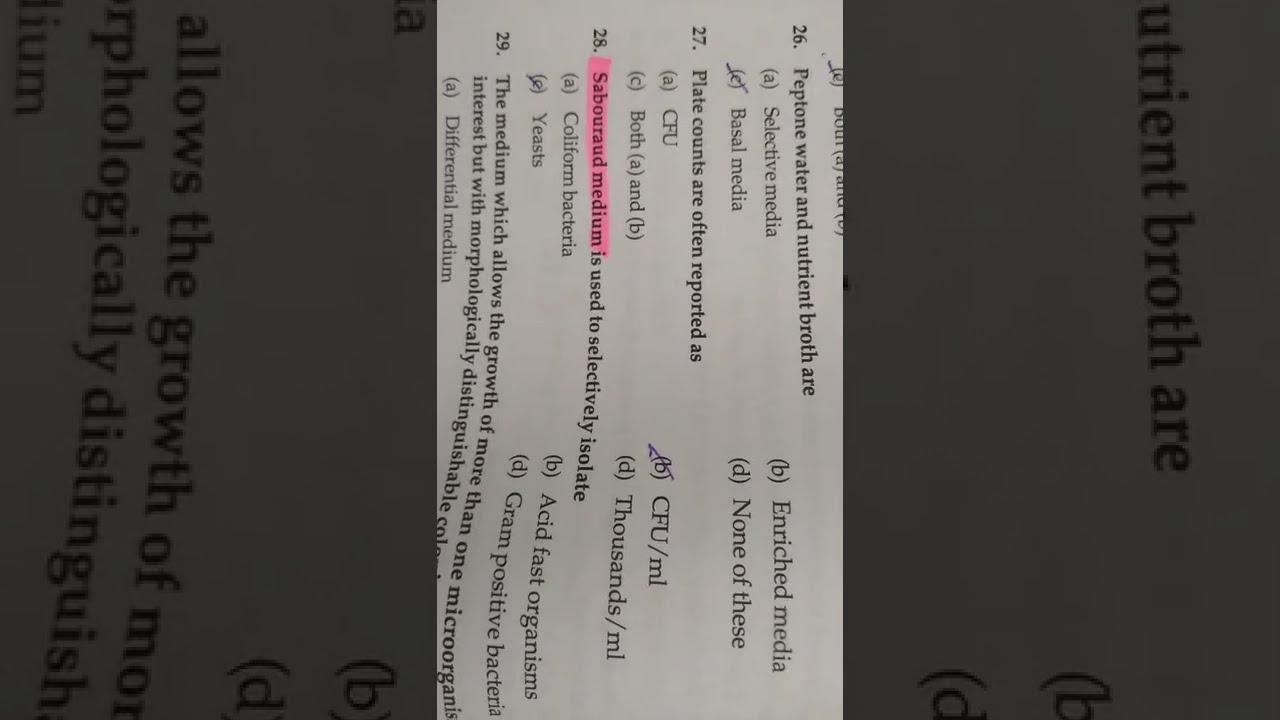The image showcases a horizontally rotated photo of a slanted test paper containing four multiple-choice questions, numbered 26 to 29, in bold black text on a white background. The questions, positioned along the left-hand side of the page, are accompanied by dark black text. Question 26 reads, "Peptone water and nutrient broth are?" with four choices: A) Select media, B) Enriched media, C) Basal media (which is marked with a diagonal slash indicating it is the selected answer), and D) None of these. Question 27, "Plate counts are often reported as?" has choices A) CFU, B) CFU/mL (marked with a diagonal checkmark), C) Both A and B, and D) Thousands/mL. Question 28 has "saborad medium" highlighted in pink and reads, "Saborad medium is used to selectively isolate?" The choices are A) Coliform bacteria, B) Acid-fast organisms, C) Yeast (marked as the selected answer), and D) Gram-positive bacteria. Question 29 is partially cropped with only part of the question visible: "The medium which allows the growth of more than one microorganism interest but with morphologically distinguishable," with only option A, "Differential medium," visible. The main image is centrally focused, flanked by zoomed-in, darker, and out-of-focus versions of the same content on the left and right sides.